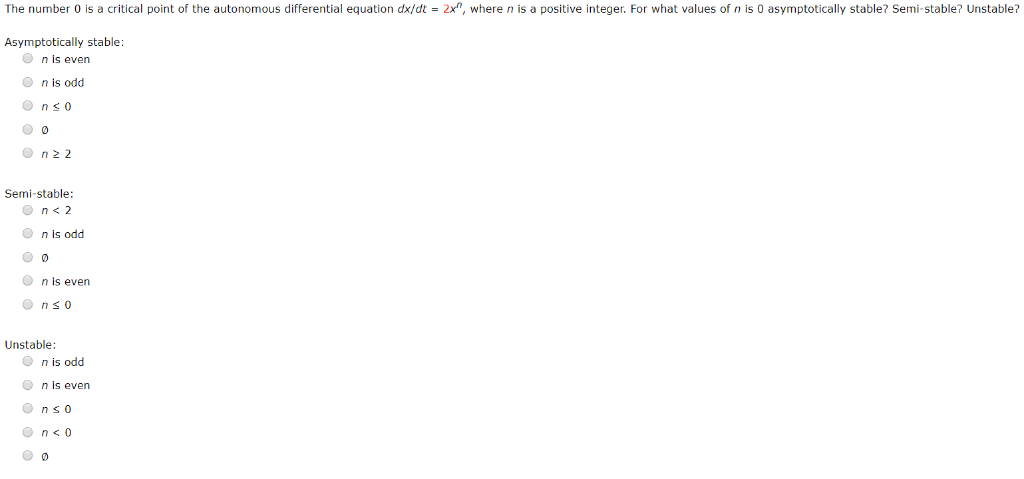The image depicts a low-resolution screenshot of a mathematical quiz interface. The entire background of the image is white, with no other UI elements visible except for radio buttons. The layout features the question at the top in a single line that stretches across the width of the image. The question, which reads "The number zero is a critical point of the autonomous differential equation where n is a positive integer. For what values of n is 0 asymptotically stable, semi-stable, or unstable?" spans the top portion of the screen. Below the question, the white space dominates most of the image with the answer options aligned along the left side.

The answer section is divided into three categories: "Asymptotically Stable," "Semi-stable," and "Unstable." Each category has a header followed by five radio buttons, presumably representing different values of n that can be selected. The radio buttons are grouped vertically under each header, and none of them appear to have been selected, indicating that this is a screenshot of the test in its initial state, without any answers filled in. The overall appearance and structure suggest a focus on determining the stability of the critical point in the differential equation through user interaction with the radio buttons.